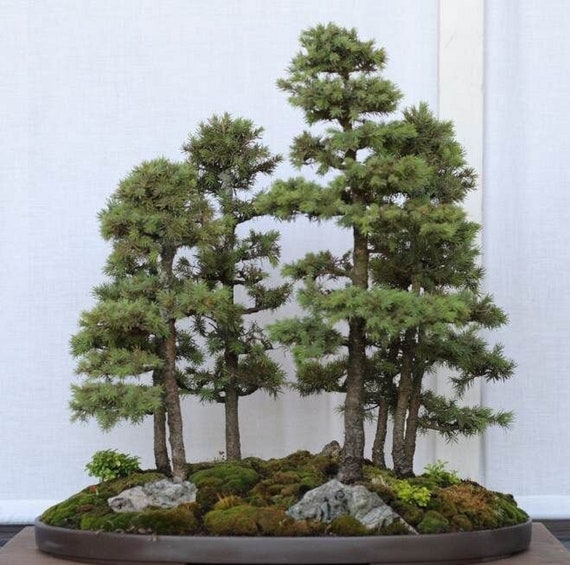The image depicts an intricate diorama, akin to a zen garden, which artistically simulates a scaled-down forest scene. Positioned atop a large, brown dish-like base, the composition features what appear to be miniature evergreen trees, reminiscent of bonsai but styled to mirror larger forest trees. There are approximately seven trees of varying heights, including one exceptionally tall tree near the center. The trees are adorned with light green leaves, suggesting a vibrant, yet realistic appearance.

Beneath these trees, the base is covered with green moss interspersed with small bushes in different shades of green and brown, mimicking natural undergrowth. Clustered amidst this greenery are scaled-down boulders, varying in color from white to gray, adding to the realism of the scene. The backdrop of the diorama is a plain white, which contrasts with the greenery and enhances the overall decorative appeal. This meticulously crafted model, likely a piece of home decor, combines organic elements with artistic design, blurring the lines between natural and artificial.